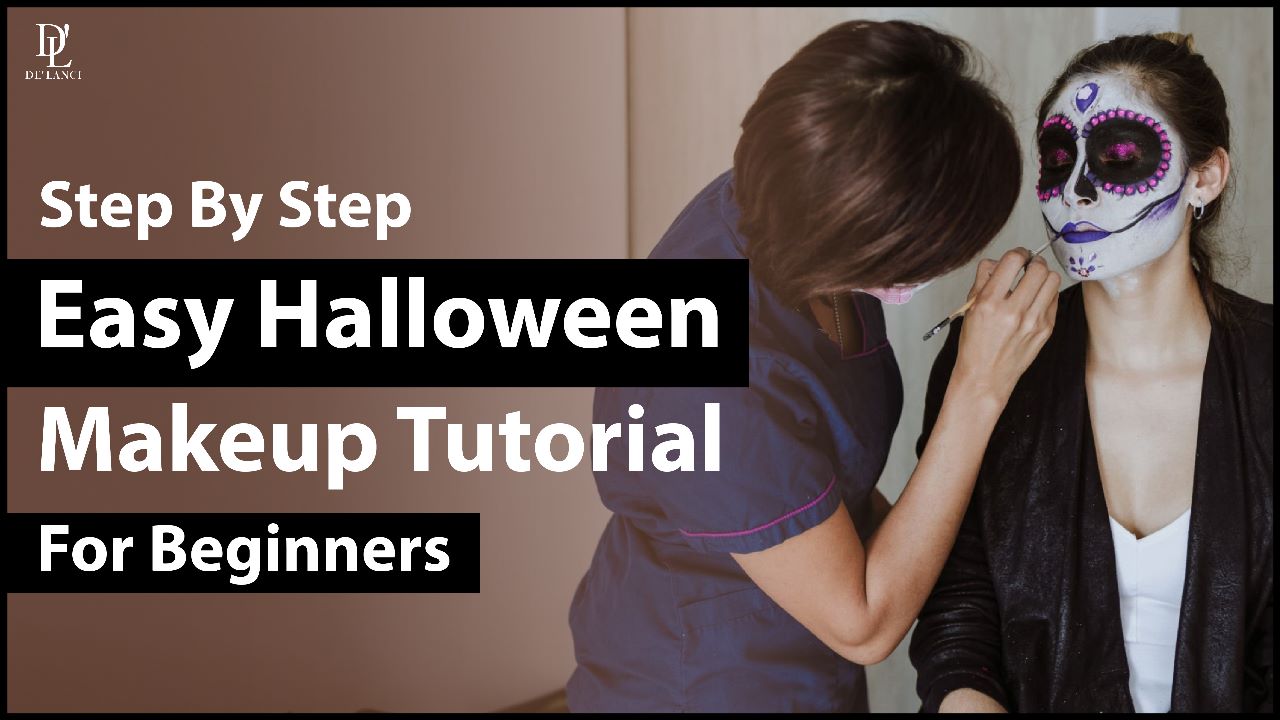This image captures a detailed step-by-step, easy Halloween makeup tutorial for beginners. In the top left corner, the logo with initials "DL" introduces the tutorial. The tutorial headline features: "Step-by-Step Easy Halloween Makeup Tutorial for Beginners," with alternating black and white text on a black background. 

On the left side of the image, the makeup artist wears a dark blue shirt with a pink-lined sleeve. She is seen in profile, meticulously applying makeup to the person on the right. The artist uses a utensil to sketch out intricate facial details.

The person receiving the makeup has their hair tied back and is wearing a black jacket over a white V-neck shirt. She is viewed from the front. Her face is predominantly white, creating a stark canvas for the Day of the Dead-inspired makeup. Large black circles cover her eye areas, encircled by pink decorations. Her lips are painted a striking purple blue. The background shifts from a light gray to a more light purple hue toward the left side of the image, enhancing the thematic Halloween atmosphere.